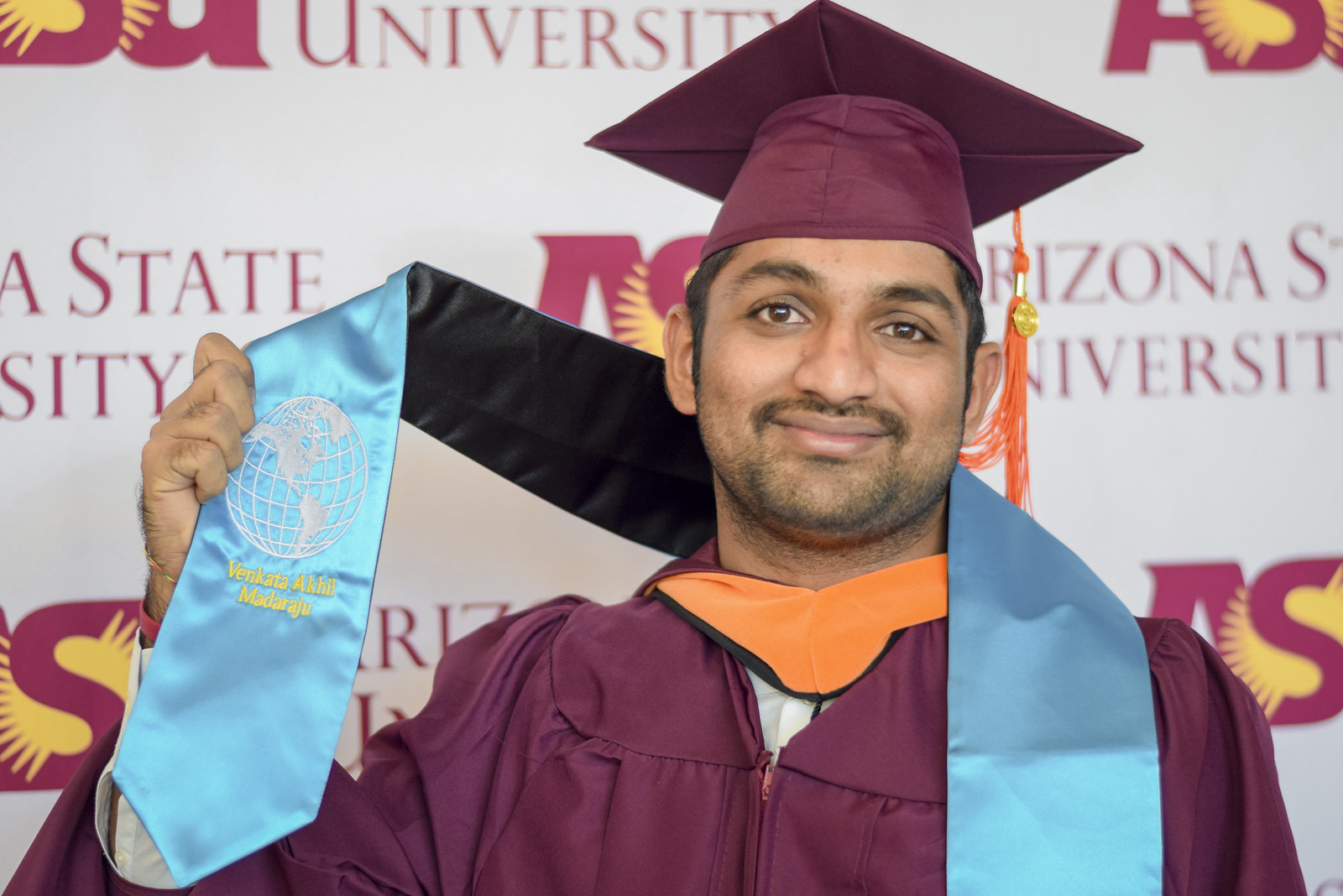The image captures a celebratory moment of a young man, Venkata Akhil Madaraju, who is proudly posing in his maroon graduation cap and gown, adorned with an orange tassel and a matching orange hood around his neck. He is standing in front of a banner that signifies his accomplishment from Arizona State University, with visible logos in maroon and yellow, the school colors. The young man, with brown skin, dark eyes, a mustache, and a light beard, beams a wide, closed-mouth smile as he holds up a satiny blue sash. The sash, draped around his neck, features an embroidered white globe and non-English lettering beneath it.